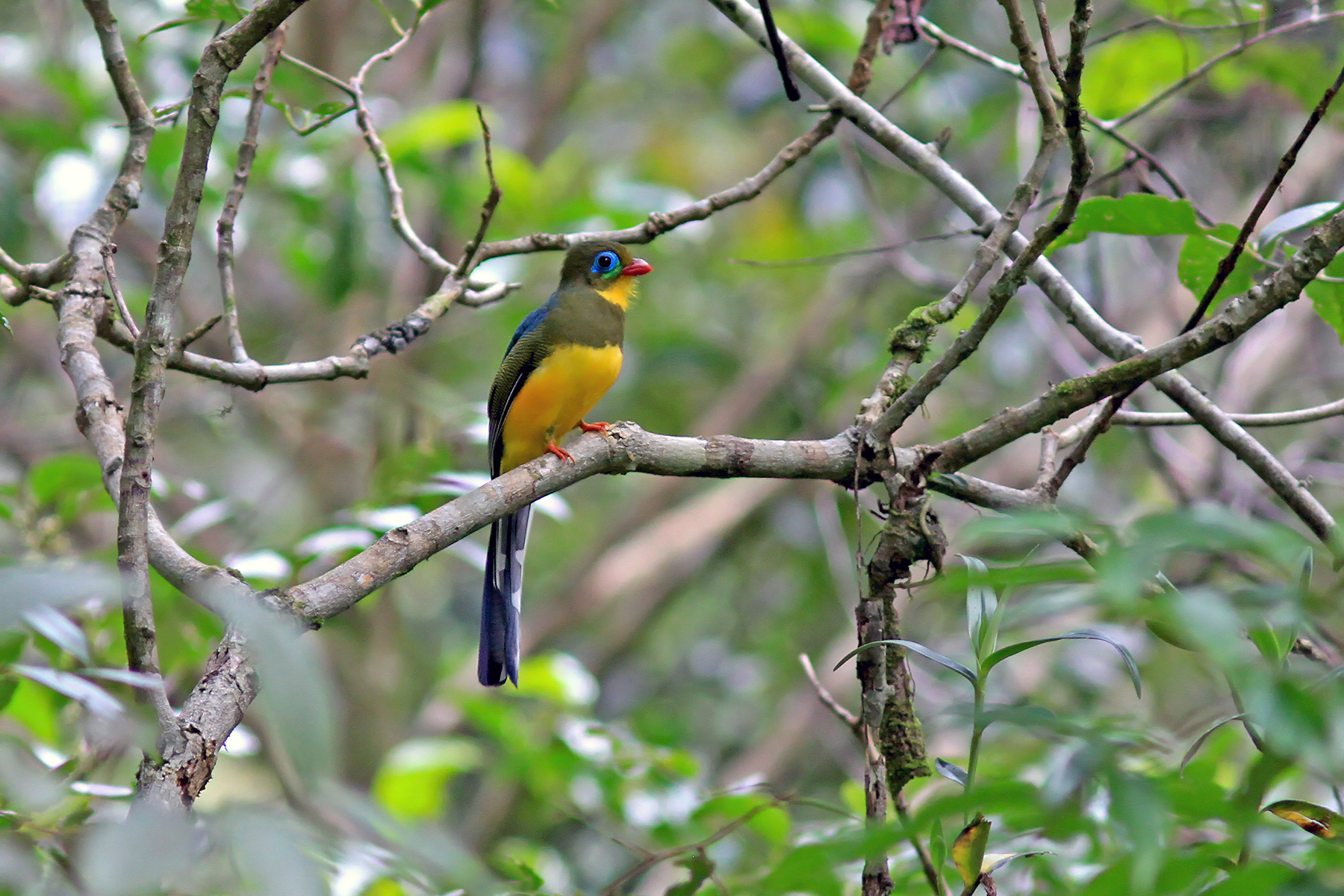In this close-up nature photograph, a vibrant tropical bird is perched on a sparse tree limb, surrounded by blurred leaves and branches in the foreground. The bird stands out with a striking array of plumage: it has a long, dark blue tail feather, a yellow abdomen, and a chest that transitions from yellow to olive green up to its head. Around its eye is an intense blue, and its beak is small and red. The bird’s back features a bright blue patch, and its claws are dark orange. The branches of the tree are light brown and devoid of leaves, creating a stark, natural backdrop for this colorful, solitary bird.